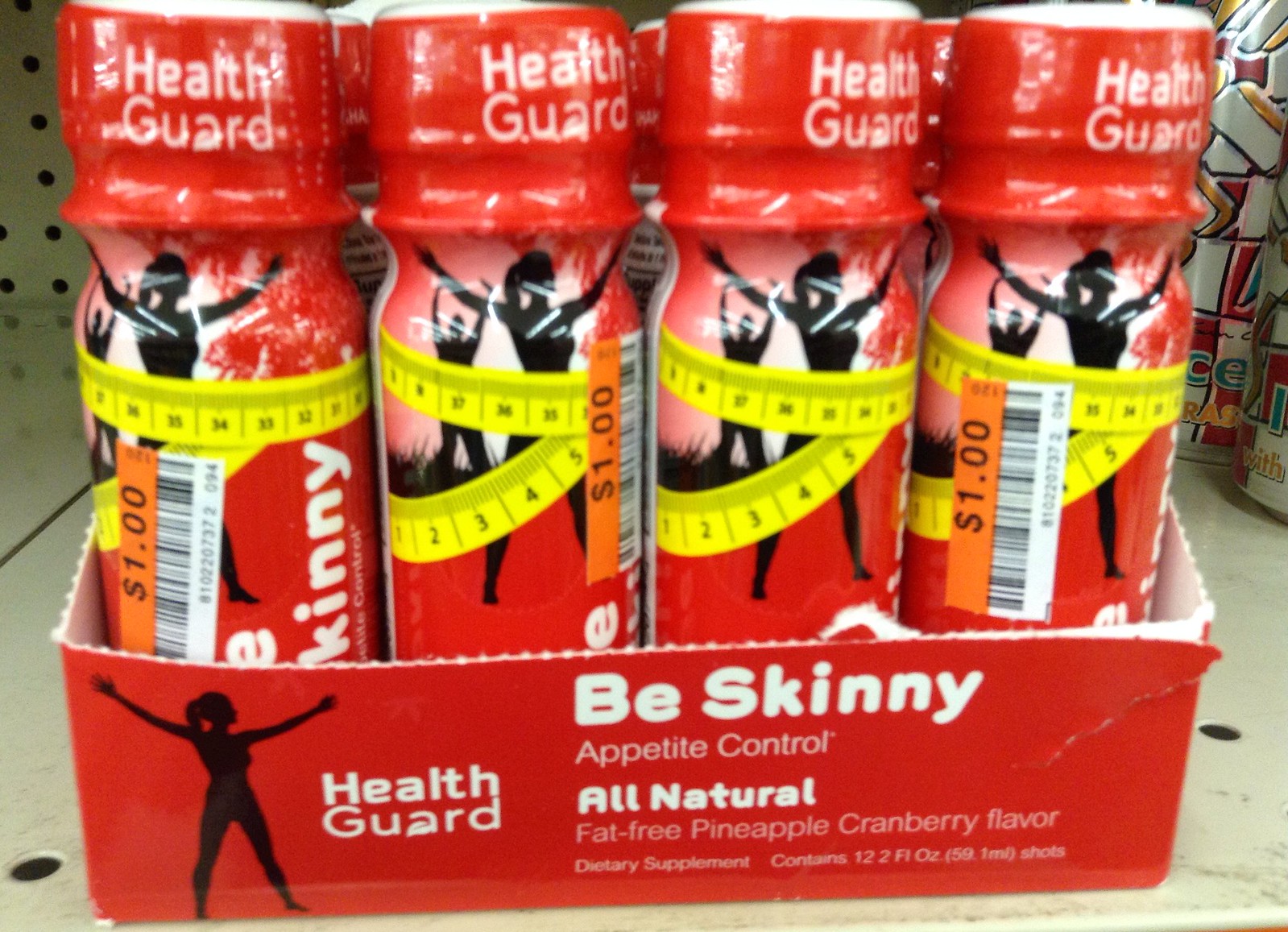This photograph, taken inside a grocery store, focuses on a shelf displaying a multi-pack of Health Guard beverages. The product is prominently packaged in sleek red bottles adorned with a yellow measuring tape design. Each bottle is labeled "Be Skinny," emphasizing appetite control, all-natural, fat-free, and boasts a pineapple cranberry flavor. It's a dietary supplement presenting 12.2 fluid ounces per shot. The packaging also features silhouettes of people, including a woman with a ponytail and a man, both depicted stretching or dancing. This multi-pack, enclosed in a box cut halfway and holding six bottles, is marked down to $1 each, as indicated by an additional label with a barcode. In the background, more of these products can be observed stacked on the beige shelf.